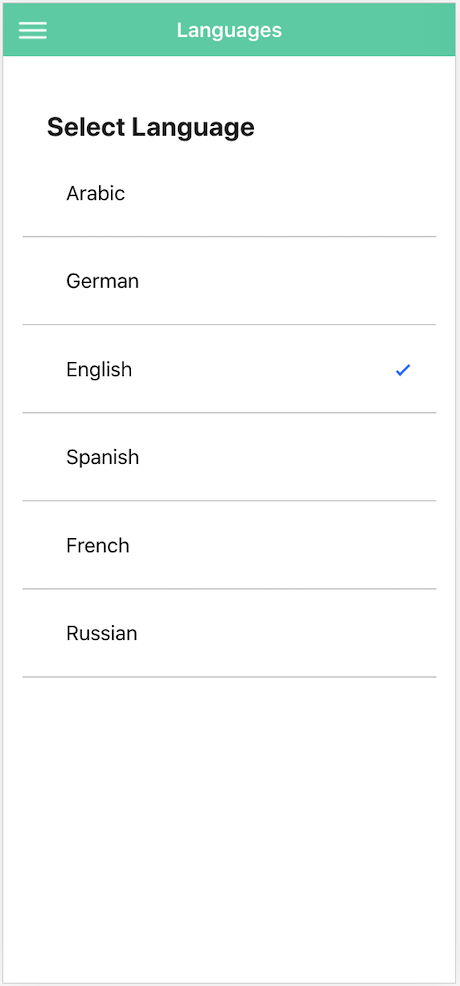This image is a screenshot of a mobile phone interface, featuring a tall and narrow rectangular page with a green header at the top. The header is decorated with three horizontal lines in white, stacked one above the other, positioned in the top left corner. Centered within this green border is the word "Languages" printed in white.

Below the header, on a white background, the page displays the text "Select Language" in large, black font. The language options are listed sequentially in black text, each separated by a horizontal line that extends across the page. 

The listed languages, in order, are:
1. Arabic
2. German
3. English (marked with a checkmark on the far right)
4. Spanish
5. French
6. Russian

The checkmark denotes that English is the currently selected language. The remainder of the page is plain white, devoid of any additional text or logos.